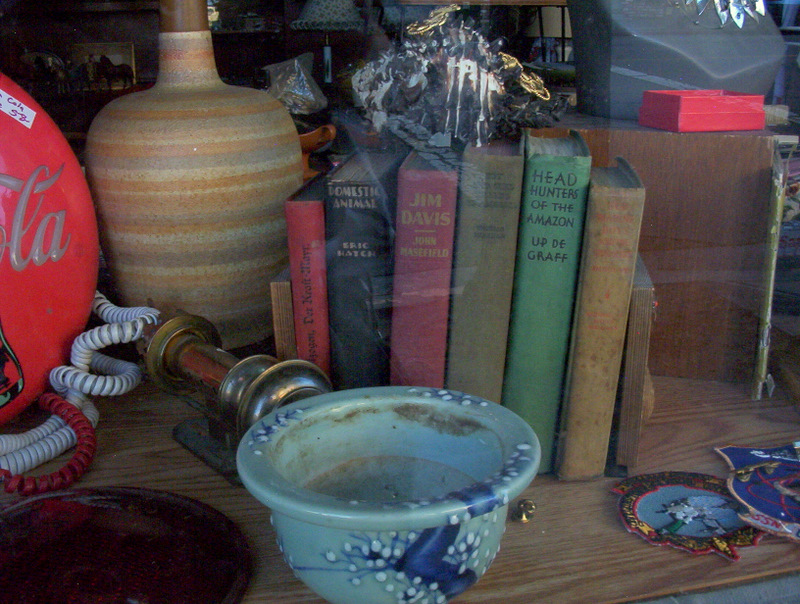The image is a detailed close-up of various items displayed in what appears to be a storage room or potentially a yard sale setup. Dominating the foreground is a wooden table with a distinct wood grain, and upon it, there's a blue-colored bowl, possibly made of ceramic or plastic, with a pipe sticking out of it that resembles a marijuana pipe. To the right of the bowl, near the top right corner, are some homemade-looking metal coasters. Behind the bowl, there's a row of old hardcover books positioned between bookends. Titles include "Jim Davis," "Headhunters of the Amazon," and "Domestic Animal by Eric Retsch," among others.

To the left of the books is a large, tan, brown, and orange vase, or perhaps the base of a lamp, with its top part cut off in the image. Adjacent to this vase-lamp, on its left side, is a tangled, white and red telephone cord typical of old-style house phones. There is also a vintage Coca-Cola sign, partially cut off in the frame, and half-hidden. Additionally, the bowl seems to have military patches, possibly naval unit patches with "SSN" indicating submarine service, which could suggest that the setting is a veteran's home. Overall, the assortment of items—military patches, vintage phone cords, old books, and an antique-looking scoop—gives the impression of a well-loved collection of antiques and memorabilia.